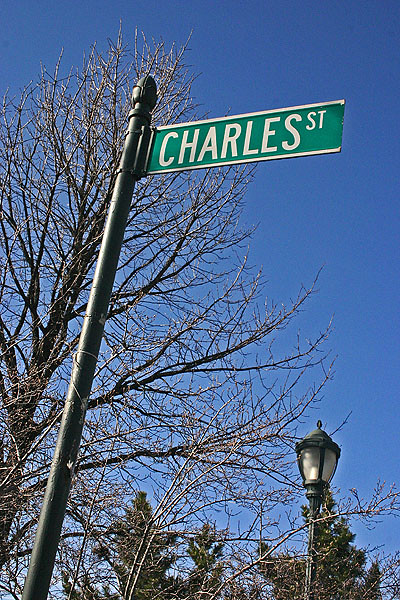A close-up photograph captures a street sign mounted on a black pole. The pole features a decorative knob at its top. The sign itself is green with white borders, displaying the word "Charles" in bold white letters. In the upper right corner, a smaller white "ST" signifies "Street". Behind the sign, a large, leafless tree extends its branches skyward, accompanied by the silhouettes of evergreen trees in the background. The clear blue sky provides a crisp backdrop, while a black streetlight with clear glass is visible in the lower right corner of the image.